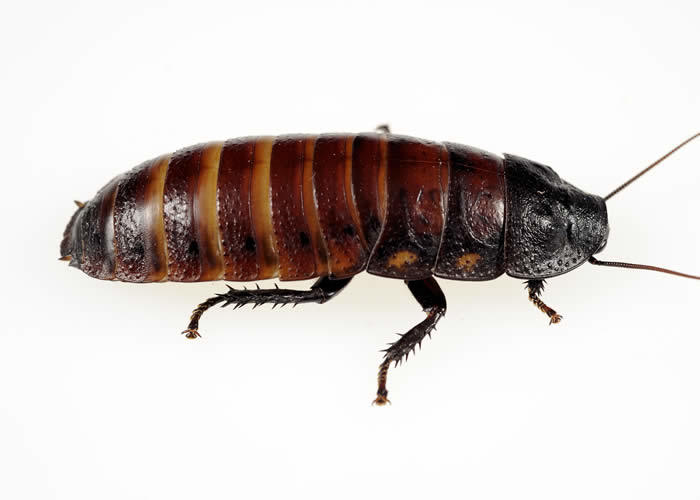The image is an indoor, close-up, color photograph of a full-grown cockroach situated against a completely white background, likely for a textbook or presentation. The cockroach occupies the entire frame, positioned horizontally with its head to the right and its tail to the left, showing a side view of its right side. Its body is segmented, featuring a brown coloration with alternating tan lines, and some yellow hues. The head is distinctly darker brown or black, with two antennae extending out of the frame, giving the impression of continuation beyond the image borders. The legs, visible and three-segmented, protrude from the bottom, characterized by spikes and pads closer to the feet. The cockroach's textured body showcases a shiny surface, adding to its detailed and striking appearance.